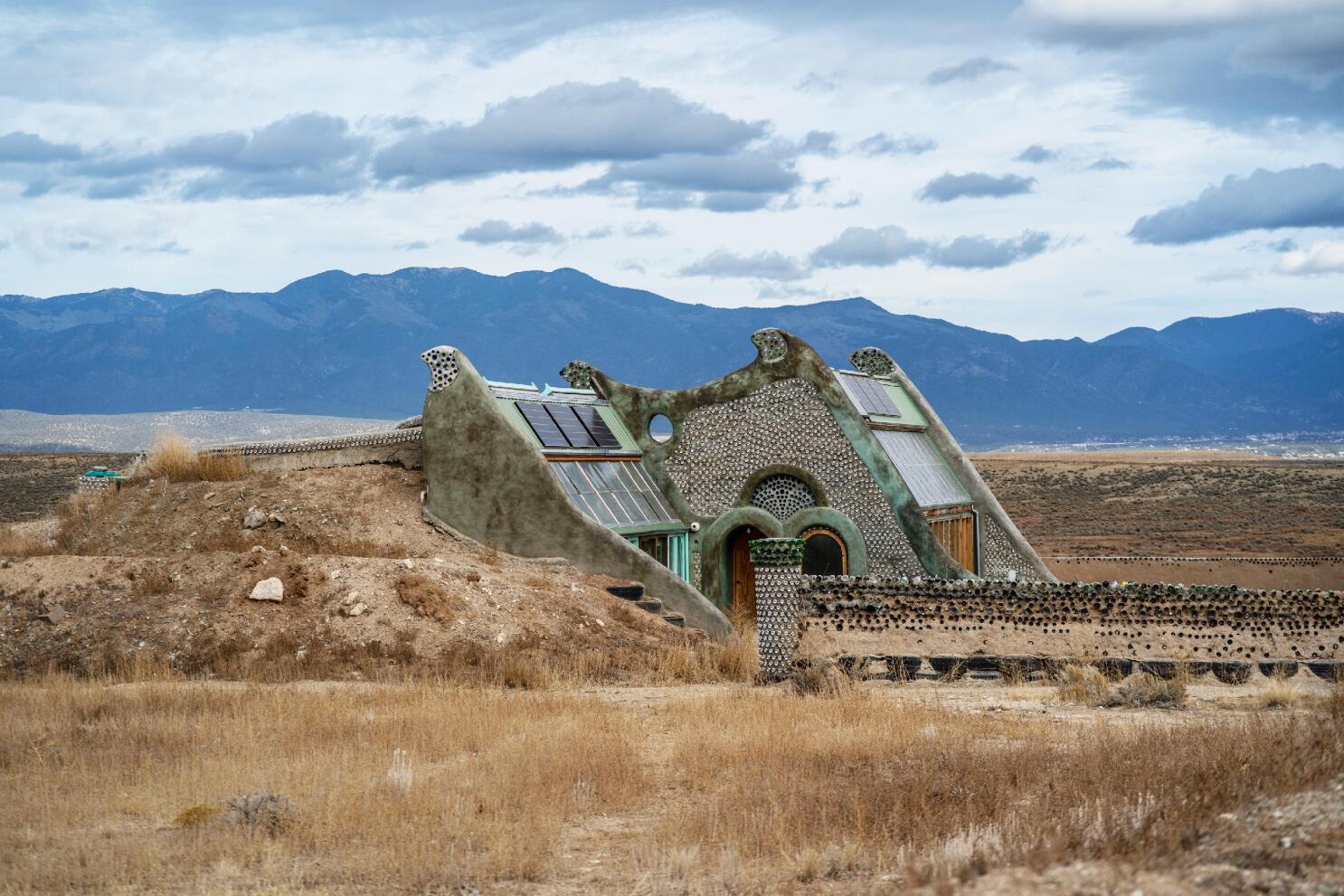This photograph captures a remarkably unique house built into the side of a large gray and tan dirt mound, blending seamlessly into its natural surroundings. The irregularly-shaped structure, reminiscent of a trapezoid, prominently features a front facade jutting out from the mound. The sky above is a cloudy blue-gray with large, puffy clouds visible, and the landscape around the house is barren, with no other buildings in sight, only dried grass and dirt hills. 

The house itself is adorned with a striking combination of materials: black and white tiles cover its exterior walls, accented with dark green trim. The house features light brown, natural-looking wooden doors and multiple square-shaped black solar panels affixed to its sides, optimizing energy efficiency. A low stone wall matching the house's design, capped with black and dark green tiles, extends from the center of the image towards the right, enclosing the property. 

Additionally, there are stone archways and steps integrated into the design, leading to various entrances, adding to the home's intricate and decorative appeal. The overall scene combines the rustic rawness of the hillside with the captivating, eco-friendly architectural details of the house, creating a unique blend of natural and built environments.